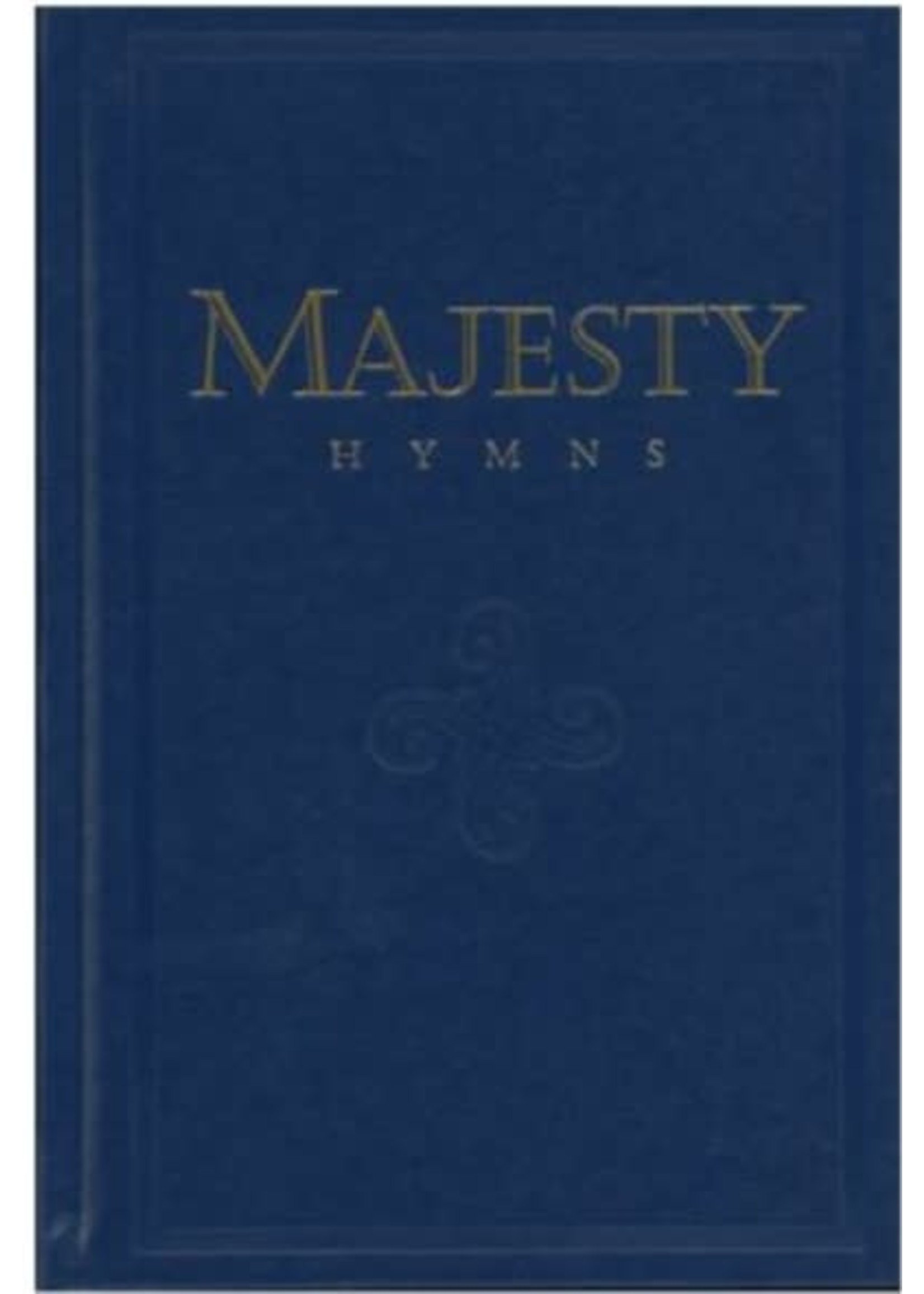The image is a detailed scan of the front cover of a "Majesty Hymns" book, presumably a church hymnal. The deep navy blue, possibly leather, hardcover prominently displays the title "MAJESTY HYMNS" in gold capitalized letters, with "MAJESTY" in a much larger font than "HYMNS." Centrally placed just below the title is a stylized emblem resembling a thick plus sign with each arm curved to the left, imprinted in the same blue color as the background, giving it a stamped or embossed appearance. The cover features a decorative, indented frame, with a narrower margin on the top, bottom, and right edges, roughly a centimeter in width, and a wider margin, about two to three centimeters, along the left edge where the spine is located. The book cover itself is viewed against a plain white background on a computer screen, emphasizing its details.